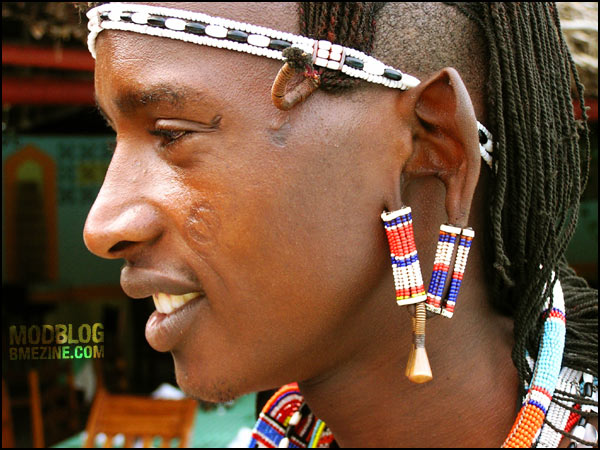This captivating close-up image features a handsome young black man in his 20s or early 30s, possibly from Africa. He is looking sideways, revealing a detailed profile that showcases intricate jewelry and tattoos. His earlobes are uniquely split into two separate sections, each adorned with long, braided, and beaded earrings wrapped in red, white, blue, and orange, featuring a gold tip. He also wears a matching necklace with orange, white, and blue beads. A headband with a tribal black, white, and blue pattern adorns his forehead, keeping his dreadlocked hair, partially shaved above the ear, neatly pulled away from his face. Text on the left side of the image reads "modblog.com," and a faint branding tattoo or scar is visible on his upper left cheek. His overall appearance, including the tribal jewelry and headband, hints at his cultural heritage.